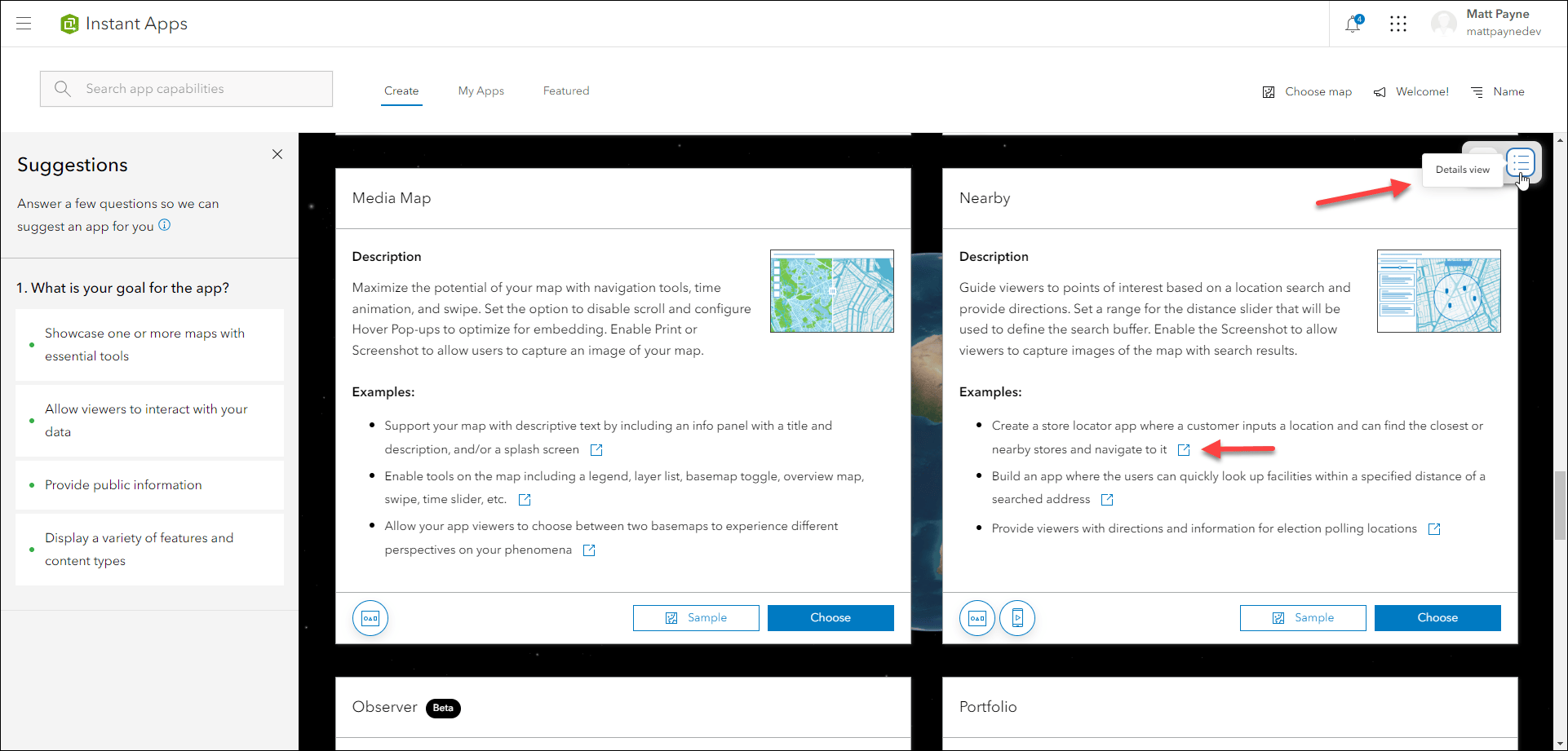The image depicts the user interface of a site named Instant Apps. In the top left corner, the Instant Apps logo is prominently displayed, featuring a small green hexagon accompanied by the name "Instant Apps" in greyish-black text. On the top right corner, there's a notification bell icon and an account access icon, indicating areas for alerts and user profile management.

Beneath these elements, a search panel is situated on the left, with multiple headings spread across the top of the screen. These headings include "Create," "My Apps," "Featured," "Choose Map," "Welcome," and "Name." Running down the left-hand side of the interface are a series of prompts aimed at guiding users, such as suggestions under "What is your goal for the app?" with several bullet-pointed reasons listed for creating an app.

Dominating the center of the screen are examples of new app creation approaches, reflecting the selection of the "Create" heading. In the left section under "Create," there is a category named "Media Map," which includes a description, examples of usage, a sample app, and a prominent blue "Choose" button for users to proceed. Similarly, on the right section, there is another category named "Nearby," equipped with its own description, examples, sample app, and "Choose" button, offering another avenue for app creation.

The image suggests a user-friendly platform providing pre-configured app templates like "Media Map" and "Nearby" for quick app development, reconfiguration, and customization, allowing users to efficiently create their own applications based on given examples and tools.